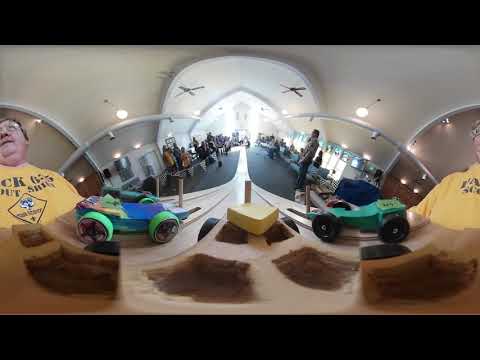The image captures an immersive view of a lively model car racing event in a spacious indoor venue with an arched roof illuminated by bright lights. At the centerpiece, a long wooden track slopes upward toward the camera's foreground and then descends through the room's center, flanked by spectators who might be part of different teams. The track is raised on wooden poles and converges into one lane as it extends through the watching crowd.

In the forefront of the image, two competitors stand on either side of the track. Both are wearing yellow shirts, though the one on the left has a distinctive diamond-shaped design with a logo, while the one on the right's shirt is plain yellow. The person on the left, who has glasses and a double chin, is looking ahead with notable focus. 

The two model cars, ready at the top of the ramp, are clearly detailed. The car on the left sports a blue body with circular green wheels and resembles a simple block of wood. In contrast, the car on the right is more aerodynamic with a cone-shaped, square-like body, black wheels, and a design reminiscent of an F1 car. This engaging scene is bustling with energy as spectators on both sides eagerly anticipate the start of the race.